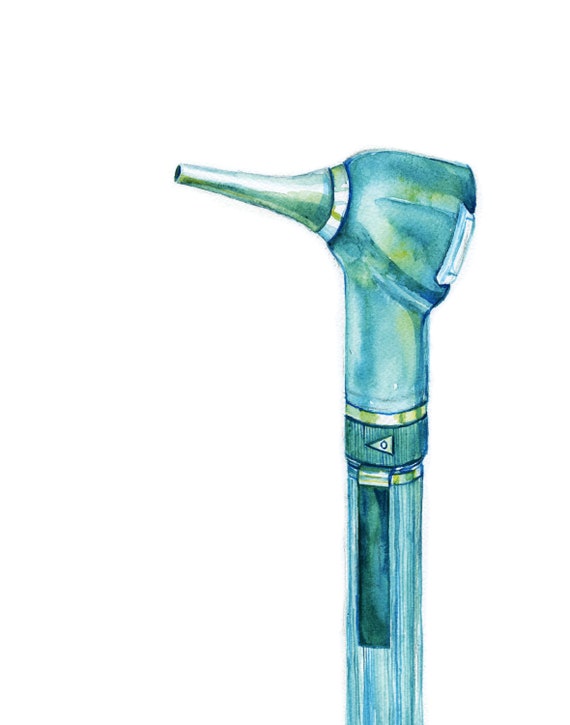The image depicts a meticulously detailed watercolor sketch of a medical instrument, possibly an ear thermometer or a stethoscope, set against a pristine white background. The primary object is a cylindrical tool rendered in shades of light teal and green. Starting at the top, there's a dome-shaped head that transitions into a cone on the left, narrowing into a small rod painted in light gray. The tool features a prominent gold band around its middle, with a dark blue vertical rectangle beneath it, which could serve as a clip for attachment. Below, the instrument continues with alternating lines of green and white, adding to its intricate design. The overall appearance is enhanced with silver accents, giving it a unique, almost trumpet-like front.